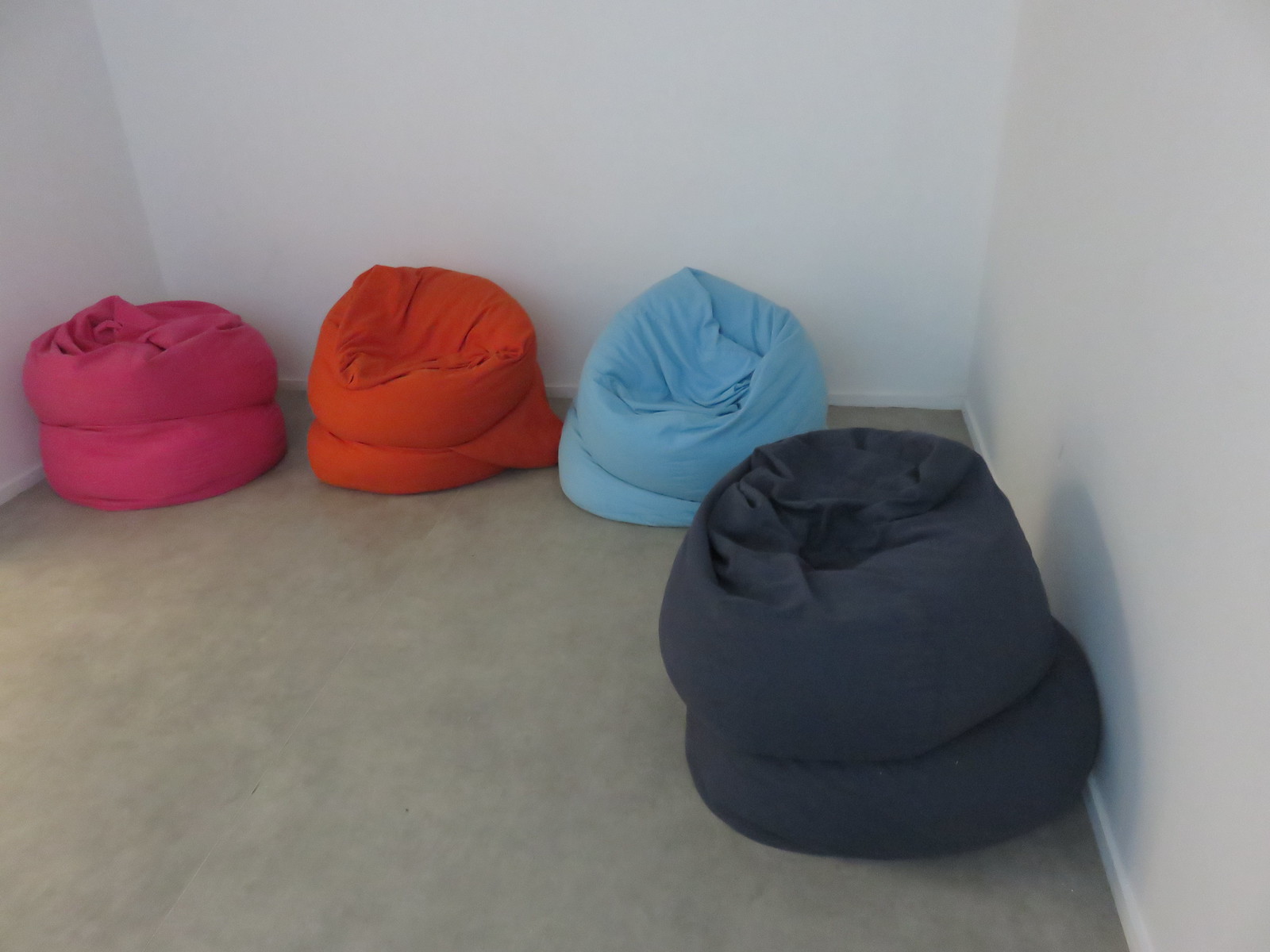The image depicts a room with three visible corners from a perspective that highlights the light gray walls and beige carpeted floor. The walls are adorned with a wooden border at the bottom. Four beanbags in varied and vivid colors—pink, reddish-orange, light blue, and black—are arranged around the room. The first three beanbags, pink, orange, and blue, are clustered together along the back wall, while the black one is positioned near a second corner, possibly near the room's entrance. Each beanbag appears double-layered with visible wrinkling and impressions on the cloth, indicating previous use, except for the black one, which remains smooth and undisturbed. The comfortable appearance of the beanbags is a prominent feature, making them seem inviting in this otherwise minimalistic setting.